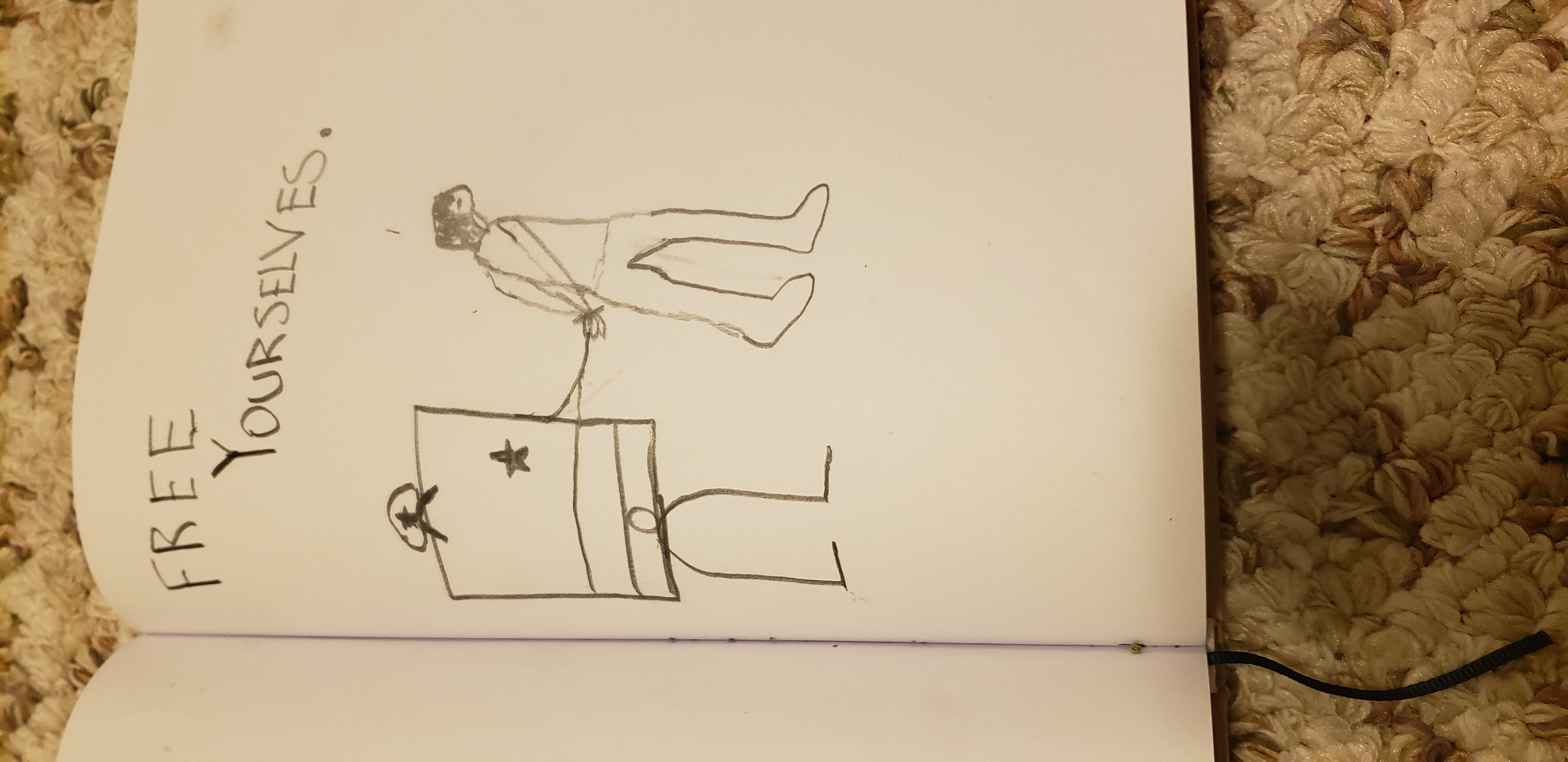A white sketch notebook is displayed on its side against a brown and tan tabletop background, rotated 90 degrees counterclockwise. The image shows the top of the notebook on the left and the bottom on the right. The open notebook presents a partial view of the left page at the bottom of the image. At the top of the page, the phrase "Free Yourselves" is written in black lettering. Below the text, a child's drawing depicts a box-bodied stick figure police officer, identified by a star on its left chest. The officer's left arm extends to handcuff or bind the hands of another stick figure, who appears to be walking away towards the top of the image. This figure's arms are drawn behind their back, their head slightly bowed. A hand or chain, seemingly originating from the police officer, is connected to the figure's handcuffs.